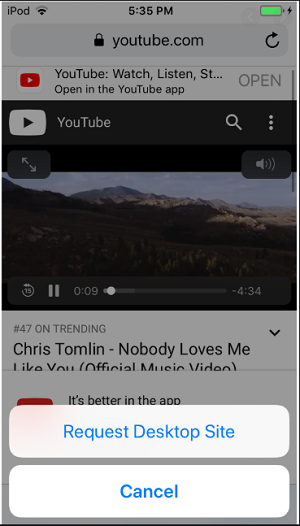The screenshot captures an iPod interface displaying a YouTube search. At the top left corner of the screen, the iconic iPod symbol is visible. The current time is positioned centrally at the top, while a bright green bar on the top right corner indicates the device's battery life. Directly beneath this bar lies the search box, where the user has entered "YouTube.com."

Below the search box, YouTube has suggested a relevant video: the official music video for Chris Tomlin's religious song, "Nobody Loves Me Like You." This recommendation likely stems from the user's previous viewing habits. 

Additionally, YouTube presents a typical advertisement at the bottom, promoting the benefits of using the YouTube app and encouraging its download. Above this ad, there are two white option boxes with blue text. One option allows the user to "Request Desktop Site," and the other provides the choice to "Cancel." These options offer the user additional functionalities while navigating the search.